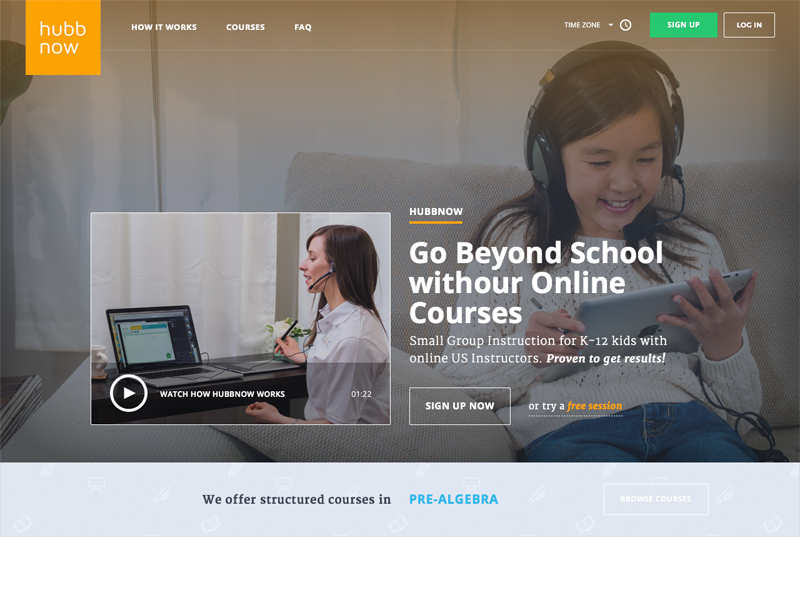This is a detailed screenshot of the home page for the "Hub Now" website, which serves as an online educational platform for small groups of children. The background features an engaging image of a young girl sitting on a couch, wearing headphones, and intently focused on an iPad. The photo is overlaid with a mostly transparent dark brown filter, adding a touch of sophistication to the design.

In the lower right corner, the site's branding "Hub Now" is prominently displayed at the top, accentuated by an orange underline. Just beneath it, a tagline reads, "Go beyond school with our online courses." Note that there is a minor typographical error, as "withR" appears as a single word instead of "with R."

Below this, additional text in white font describes the service: "Small group instruction for K to 12 kids with online US instructors proven to get results," with the phrase "proven to get results" emphasized in bold white font. Centrally located is a large white-outlined button with the call-to-action, "Sign up now," written in large white font. To its right, another option reads, "Or try a free session," with "free session" italicized in orange for emphasis.

On the left side of the screen is a large video thumbnail featuring a woman wearing a headset, seated behind a desk and concentrating on a laptop screen. At the bottom of this thumbnail is a play button beside the text "Watch how Hub Now works."